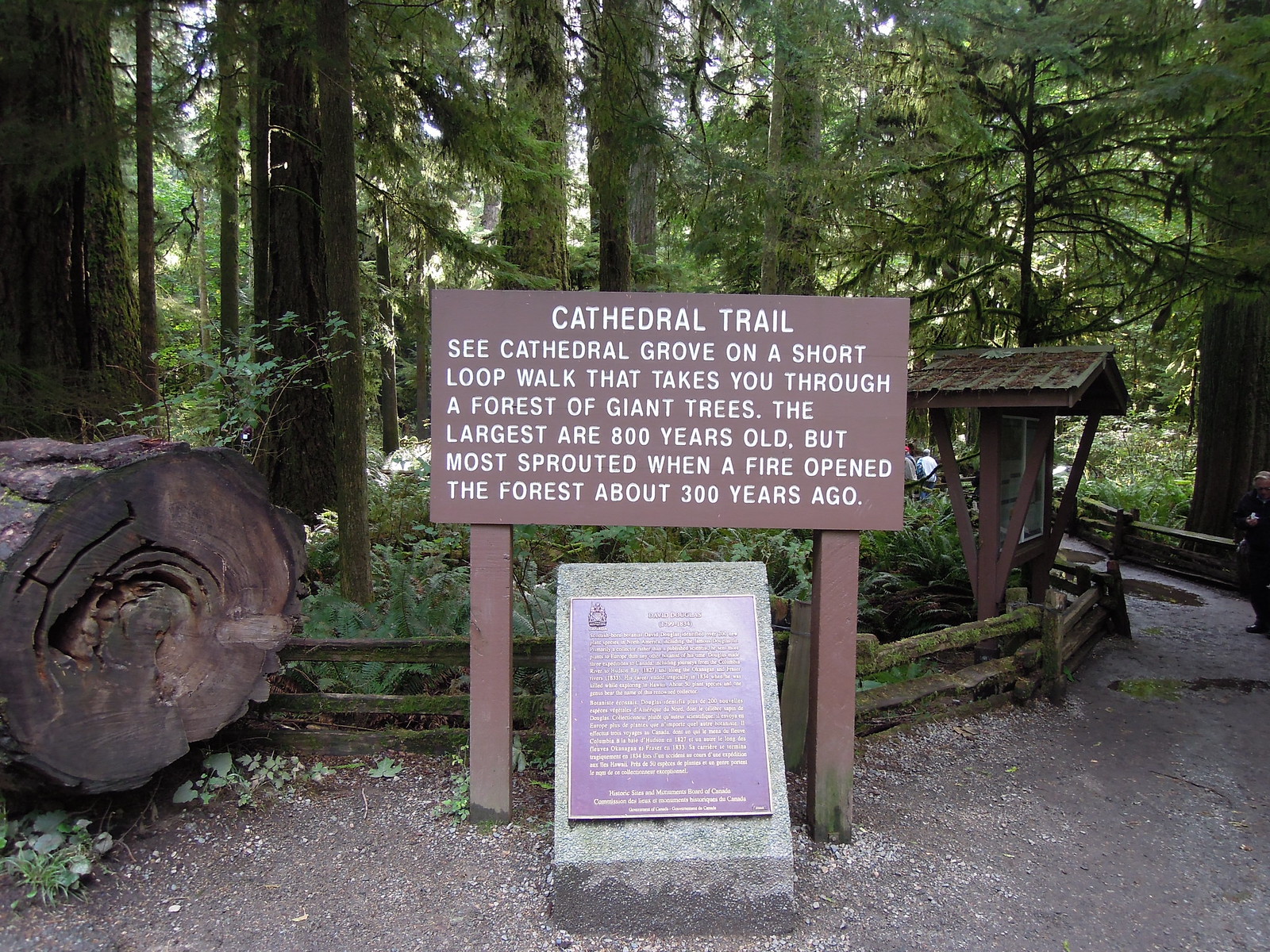This daytime outdoor photograph features a scenic walking path in a densely forested area, dominated by a central wooden sign and a plaque on a stone monument beneath it. The sign, held up by two wooden posts, reads "Cathedral Trail" in white letters, followed by a detailed description: "See Cathedral Grove on a short loop walk that takes you through a forest of giant trees. The largest are 800 years old, but most sprouted when a fire opened the forest about 300 years ago." The stone monument below the sign has a metal plaque, which partially reads "David Douglas, 1799 to 1834" and "Historic Sites and Monument Board of Canada."

Surrounding the monument is a dirt and gravel path, bordered by a low wooden fence that guides visitors through the trail. To the left of the monument lies a giant tree stump, indicative of the forest's ancient and ongoing life cycle. The scene is rich with color, showing browns and greens from the trees and foliage, alongside various shades of gray from the rocky path. In the background, a group of people can be seen in the distance walking along the path, which is enveloped by towering pine trees, adding depth and emphasizing the grandeur of the forest.